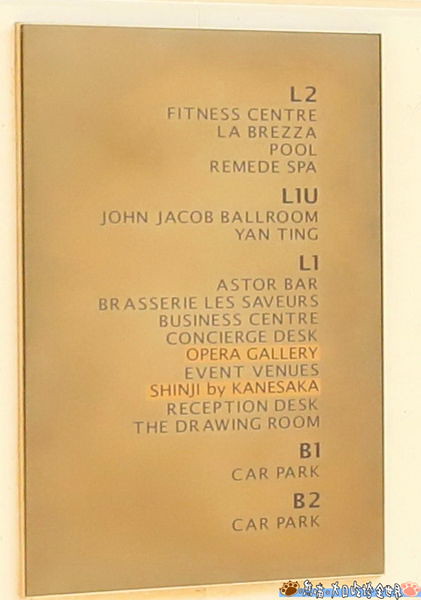The image features a close-up of an informational plaque with dark orangey-brown gold tones against a light yellow background, typically seen in a hotel or resort setting. The plaque, which has text engraved in black, details the locations of various facilities within the hotel. For Level 2 (L2), it lists the Fitness Center, La Brezza, Pool, and Remedy Spa. Level 1 Upper (L1U) includes the John Jacob Ballroom and Yan Ting. Level 1 (L1) covers the Aster Bar, Brasserie Les Saveurs, Business Center, Concierge Desk, Opera Gallery, Event Venues, Shinji by Kanesaka, Reception Desk, and The Drawing Room. Basement levels B1 and B2 are designated for the Car Park. Additionally, at the bottom right corner, there are intricate details including two paw prints—one tan with brown and the other pink—set against a blue background, flanking a series of white characters, possibly Chinese symbols.